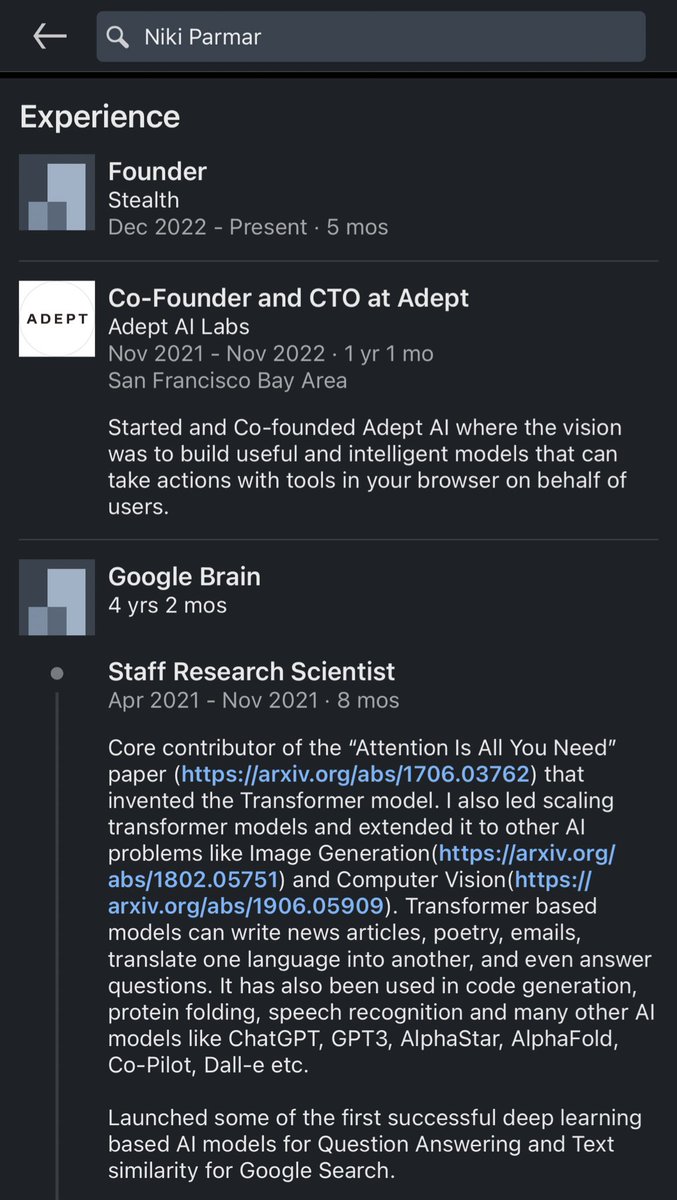The image is a screen capture featuring a predominantly black background with gray and white text. At the top of the image, there's a white back arrow and a gray search box with a magnifying glass icon. The text includes various segments detailing the professional experience of an individual named Nikki Parmer.

1. **Current Position**:
   - **Title**: Experienced Founder (Stealth)
   - **Duration**: December 2022 to present (5 months)
   - **Additional Details**: This section is marked with a gray box icon.

2. **Previous Roles**:
   - **Co-founder and CTO at Adept AI Labs**:
     - **Duration**: November 2021 to November 2022 (1 year 1 month)
     - **Location**: San Francisco Bay Area
     - **Description**: Nikki Parmer started and co-founded Adept AI Labs, aiming to develop intelligent models that can perform actions using tools within a user’s browser. This section includes a white box with the text "Adept" in black.
   
   - **Google Brain**:
     - **Duration**: 4 years 2 months
     - **Role**: Staff Research Scientist
     - **Tenure**: April 2021 to November 2021 (8 months)
     - **Contributions**:
       - Core contributor to the "Attention is All You Need" paper, which introduced the transformer model (highlighted by a blue hyperlink).
       - Led efforts to scale transformer models and apply them to broader AI problems like image generation and computer vision (each reinforced with a hyperlink).
       - Transformer-based models have diverse applications, such as writing news articles, composing poetry, sending emails, translating languages, and answering questions. They are also utilized in code generation, protein folding, and speech recognition, with applications in famous AI models like ChatGPT, GPT-3, AlphaStar, AlphaFold, GitHub Copilot, DALL·E, etc.
       - Launched pioneering deep learning AI models for question answering and text similarity within Google Search.

Notable in the image is the excellent, easy-to-read font, with minimal pixelation or blurring, ensuring clarity and legibility of the text.